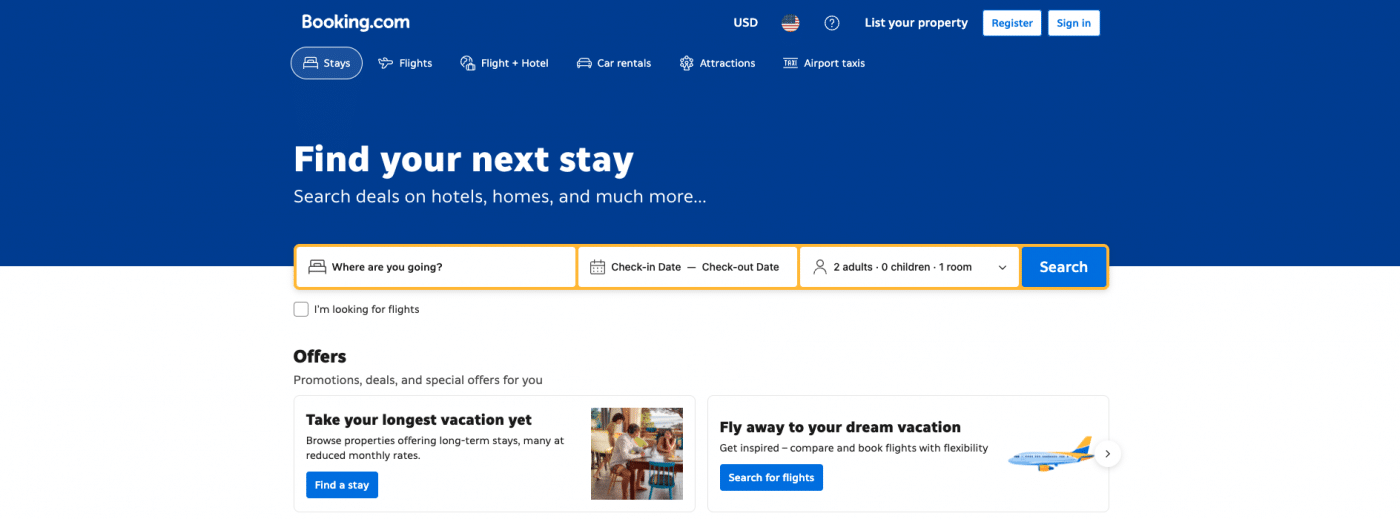The Booking.com website features a prominently large rectangular header with a dark blue background. Positioned at the top left corner in white font is the Booking.com logo. Below the logo is a navigation menu with various options, the first being "Stays," which is highlighted with a lighter blue background and a light blue oval border, indicating it is selected. The subsequent options are "Flights," "Flight + Hotel," "Car Rentals," "Attractions," and "Airport Taxis."

At the top right, bold lettering displays "USD" followed by an American flag icon within a circle. Adjacent to it is another circle housing a question mark, and next to that, in bold white text, the phrase "List your property" is showcased. Two white buttons with blue lettering follow: "Register" and "Sign in."

Beneath this section, bold white text proclaims, "Find your next stay," accompanied by a lighter white text tagline, "Search deals on hotels, homes, and much more..." Below this, there is a search field labeled "Where are you going?" with a bed icon next to it, outlined in orange. An orange divider follows, leading to a section labeled "Check-in date - Check-out date" alongside a calendar icon. To the left of this is a field displaying "2 adults - 0 children - 1 room" with a person icon and a dropdown arrow.

To the right of these fields is a search button in dark blue, adorned with white text reading "Search."